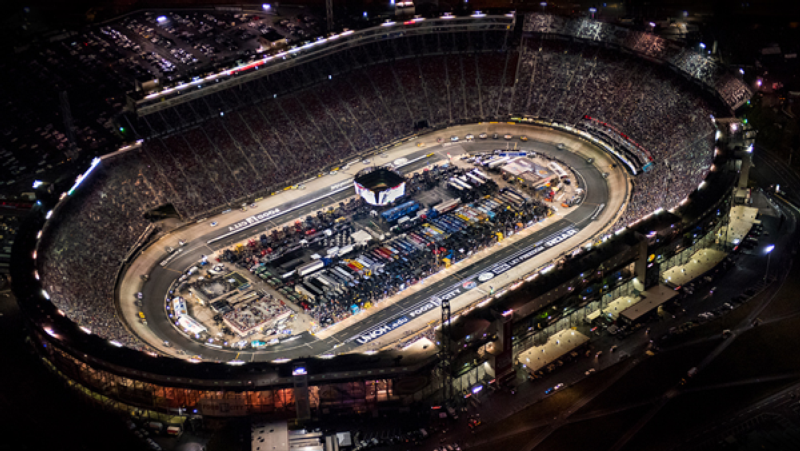This aerial nighttime photograph captures a bustling sports stadium with a racetrack at its heart. The stadium has a rectangular shape, though the oval racetrack inside garners immediate attention. The dark gray asphalt track is illuminated by a multitude of lights, accentuating the racing cars spaced along the outer edge, especially noticeable towards the top right and bottom left corners. In the center of the racetrack, a vivid array of parked vehicles, including multi-colored tractor-trailer trucks, adds a splash of color to the scene. The stadium's tiered audience seating is well-lit, revealing a large crowd of spectators. Surrounding the stadium, the darkness is punctuated by illuminated parking lots, particularly visible in the top left and bottom right corners, where numerous cars are parked. Advertisements around the track read "Union" and "Food City," contributing to the vibrant and commercial atmosphere of the event. The strategic lighting paints a clear picture of a lively racetrack event under the cover of night.